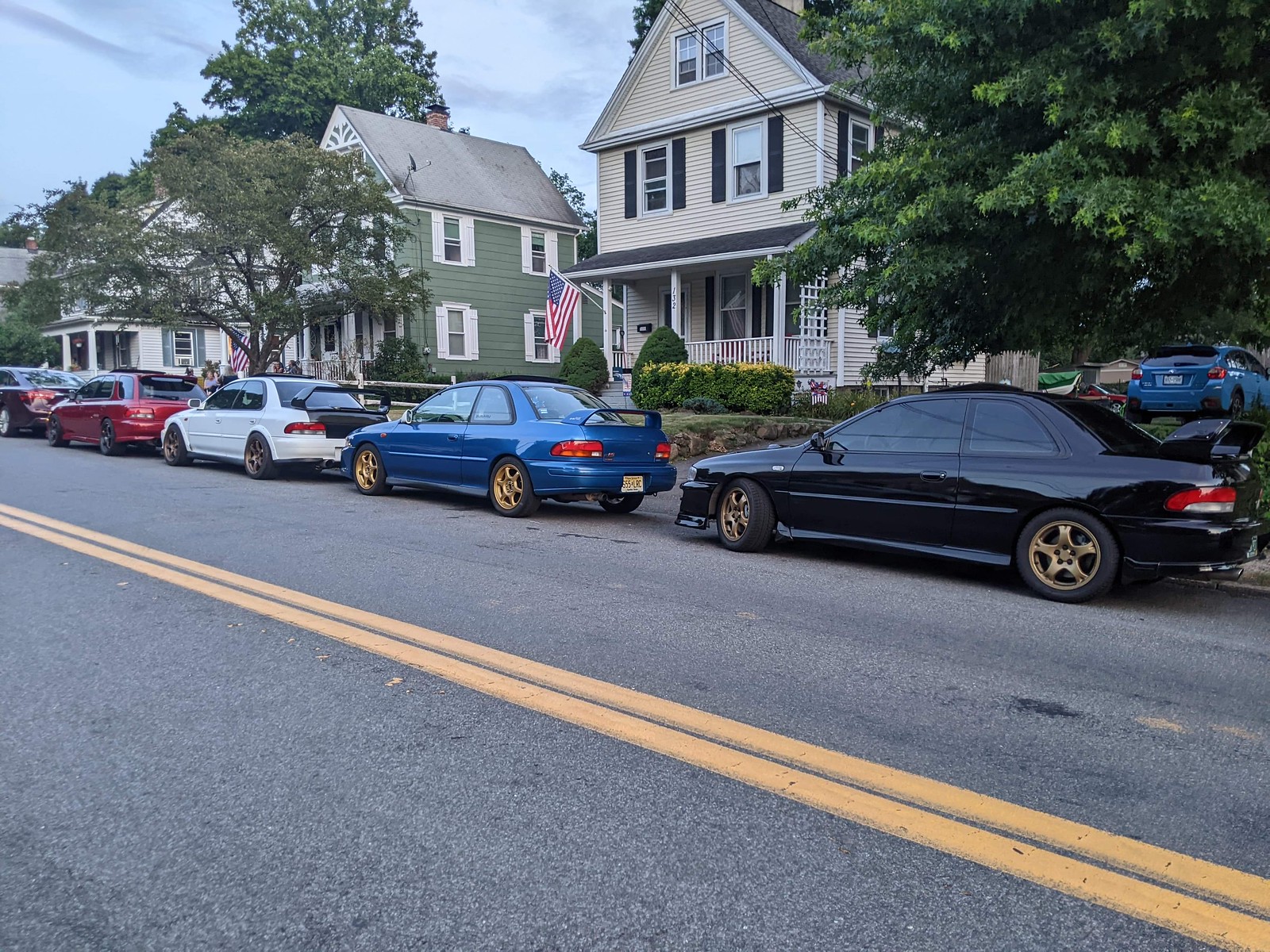This photograph captures a quintessential American residential street. In the background, three distinct houses line the horizon, all partially obscured by tall, green trees. The house on the far left is a white, single-story structure with charming blue shutters. Adjacent to it is a green house with white shutters, proudly displaying an American flag on its porch and featuring a tree in its front yard. The third house, a white two-story building, also with a porch and an American flag, stands prominently and has a large green tree to its right.

In the midground, a row of five cars is parked along the concrete street with a double yellow line running down the center. These cars include a black car at the far left edge, followed sequentially by a red car, a white four-door sedan, a blue two-door car, and another black car closest to the camera. Notably, one of the cars seems to partially block a driveway.

The street appears moderately busy, typical of an urban neighborhood rather than a secluded suburban cul-de-sac. The asphalt shows some splotches, possibly oil stains, adding to the lived-in feel. Above, the sky is a blend of blue and gray, with wispy clouds scattered throughout. The well-kept yards and overall tranquility reflect an everyday yet picturesque American city scene.